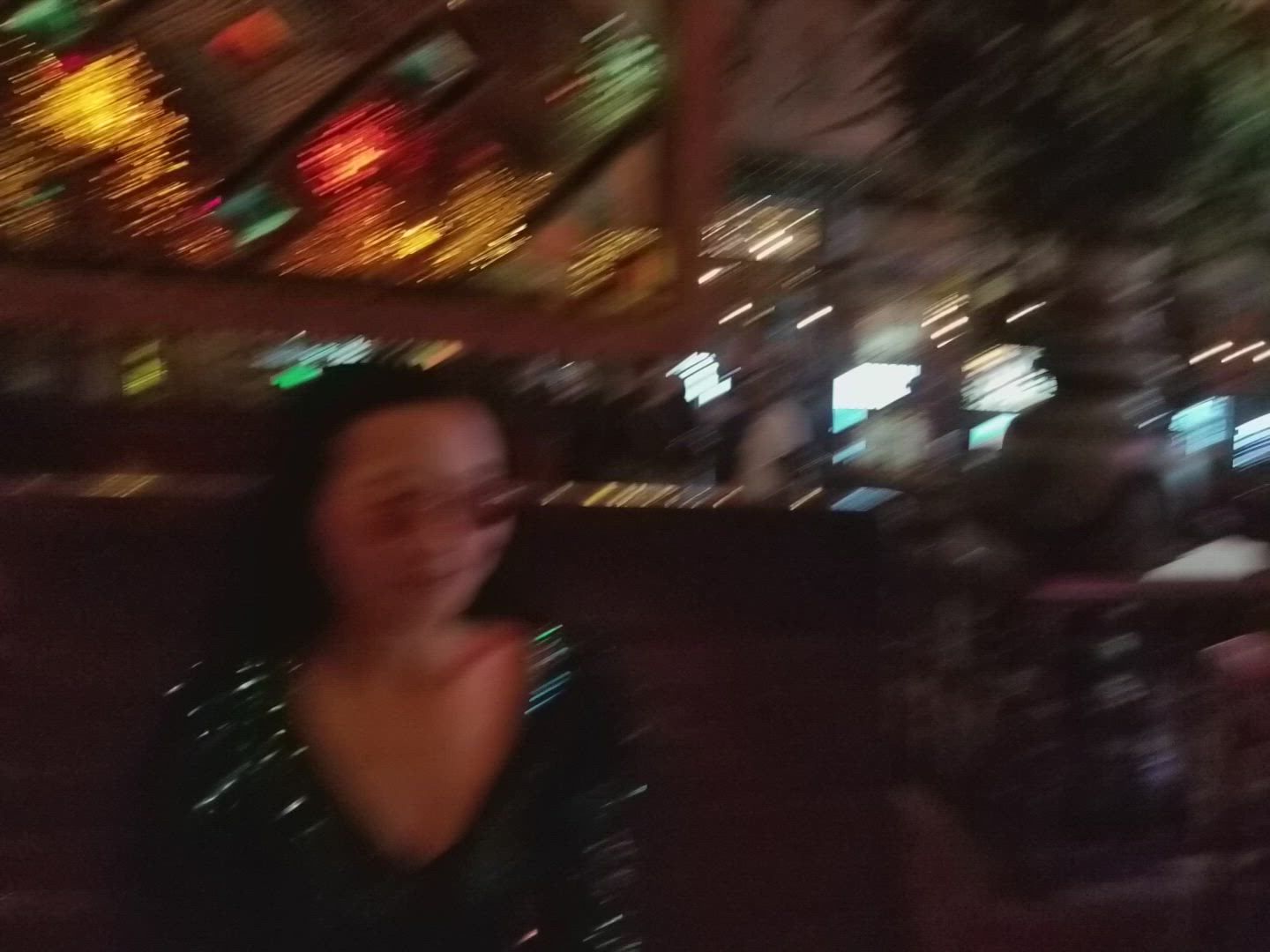The photograph, though blurry, captures the interior of a restaurant setting. At the focal point, there is a tall-backed seat made of dark brown wood. A woman with short black hair and petite features is seated against it. She has dark tanned skin and is wearing eyeglasses. Her attire appears to be formal, as she dons a v-neck top or dress adorned with striking green sparkles. The background above her head is a blur of various colors, predominantly yellow, red, and green. To her right, a tall plant resides in a cylindrical gray container, adding a touch of greenery to the scene. The background also features windows and several vertical, yellow, rectangular shapes, possibly depicting light streaming into the restaurant.